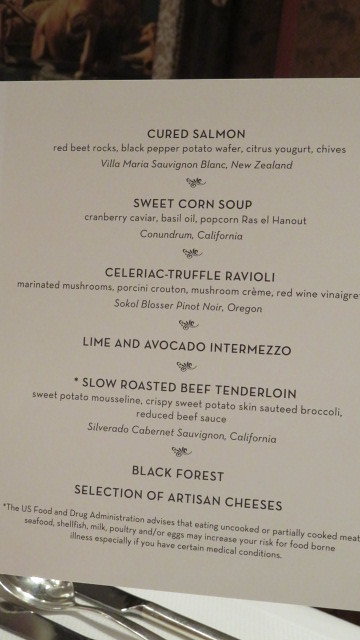This image captures an elegant restaurant setting featuring a detailed fine dining menu prominently displayed. The menu card, showcasing white text on a black background, is placed atop a white tablecloth beside a neatly set table adorned with polished silverware, including knives, a fork, and a spoon, and a folded cloth napkin. The menu lists an exquisite seven-course meal beginning with cured salmon, accompanied by red beet rocks, black pepper potato wafers, citrus yogurt, chives, and paired with a Villa Maria Sauvignon Blanc from New Zealand. Following this is a hearty sweet corn soup garnished with cranberry, caviar, basil oil, popcorn, and ross el hanout, complemented by Conundrum from California. Next is a celeriac truffle ravioli, which transitions to a lime and avocado intermezzo, then a slow-roasted beef tenderloin. The meal concludes with a black forest dessert and a selection of artisan cheeses, suggesting a lavish dining experience without listed prices, emphasizing the restaurant's upscale nature.